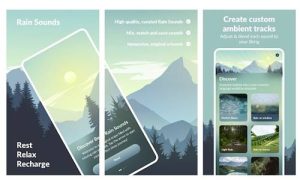This digital pamphlet presents the "Rain Sounds" app, designed to help users rest, relax, and recharge. The layout is a triptych of equally sized rectangles set against a stunning backdrop of sunlit mountains and a tranquil forest. 

The first, leftmost rectangle prominently features the app name, "Rain Sounds," along with the slogan "Rest, Relax, Recharge." An overlapping mock-up of a smartphone displays a glimpse into the app's interface, showing its sleek and user-friendly design.

The second, central rectangle contains additional descriptive text about the app, though it is slightly blurred in this image, hinting at more detailed features and benefits available within the program.

In the third, rightmost rectangle, another smartphone mock-up is showcased, featuring a collage of various natural environments. At the top of this section, bold text invites users to "Create Custom Ambient Tracks," highlighting the app's customization options for personalized relaxation experiences.